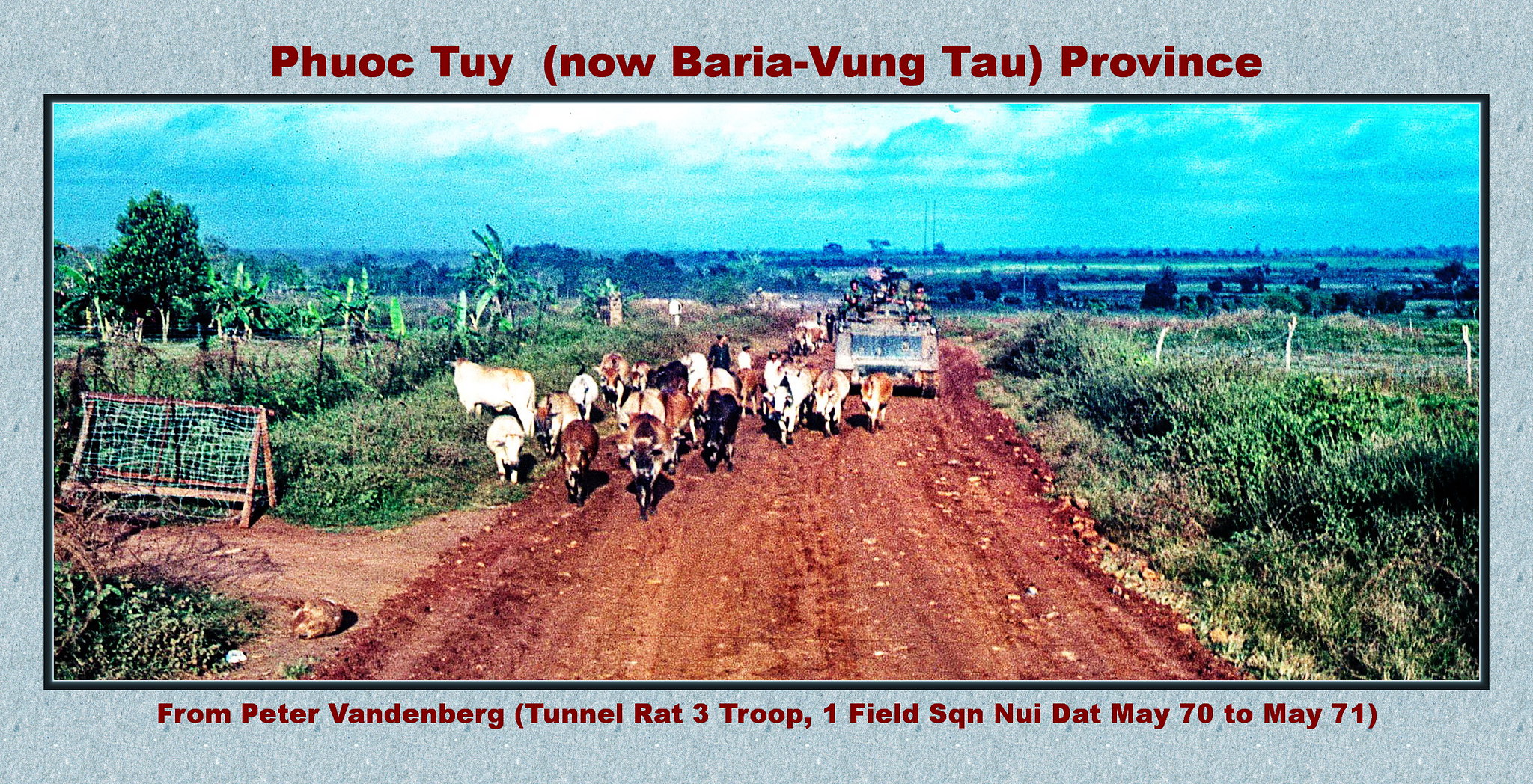This photograph captures a moment from a rural landscape, most likely during the Vietnam War, as indicated by the red text at the top that reads "PHUOC TUY (now Baria Vung Tau Province)" and a caption below noting "From Peter Vandenberg, Tunnelrat 3 Troop, 1 Field SQN, Nui Dat, May 70 to May 71." The image shows a herd of cattle of various colors—white, brown, and black—ambling down a dirt road. Flanking the road are rustic wire fences and sparse foliage, with some trees and mountains visible in the background under a cloudy sky. There are soldiers evident in the background, either walking or riding in what appears to be a tank, though it is small and somewhat difficult to discern. The presence of these soldiers suggests this photograph was taken during a military operation in a remote farmland area.